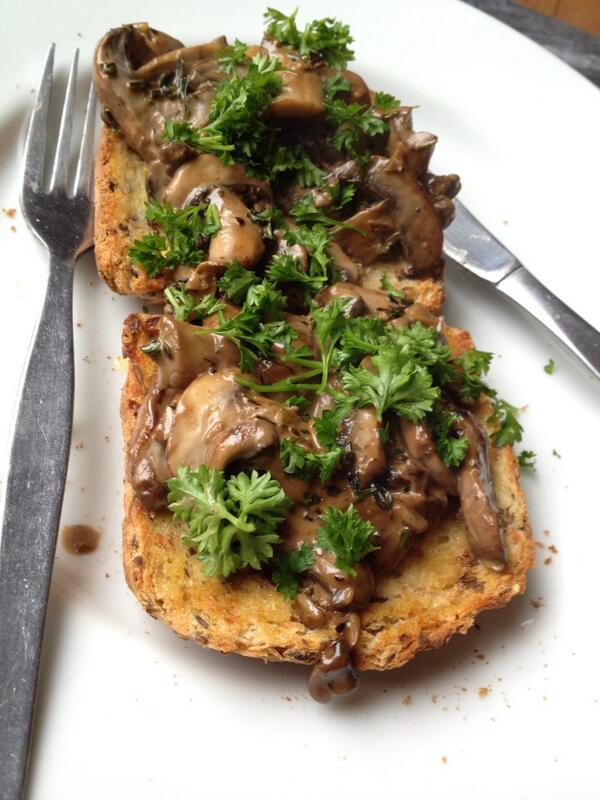On a pristine white plate, two slices of crusty Texas or garlic toast are elegantly presented as an appetizer. Each slice is generously topped with a rich, mushroom-based sauce, creating a harmonious blend of textures and flavors. The mushrooms are bathed in a savory brown sauce that envelopes them without being overly runny. This sauce clings perfectly to the toast, ensuring that each bite is flavorful and moist. Delicately sprinkled atop the mushrooms are freshly chopped green herbs, possibly cilantro, adding a burst of color and a hint of freshness to the dish. Accompanying the plate are a fork on the left and a partially obscured butter knife on the right, completing the sophisticated presentation of this tantalizing appetizer.